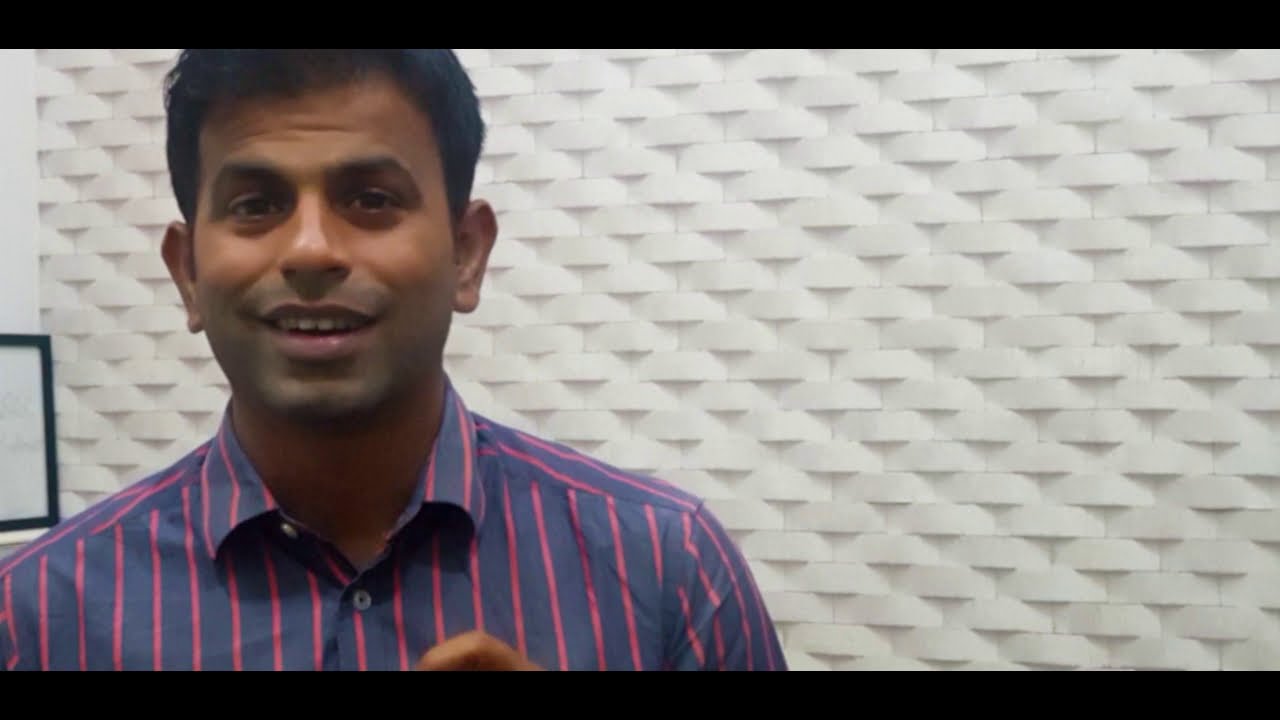The image depicts a man with brown skin, short black hair, and a five o'clock shadow, standing in front of a distinctly patterned white wall that resembles a basket weave. The man, who appears to be of Indian or Pakistani descent and roughly 35 to 40 years old, is positioned on the left side of the frame. He looks directly at the camera, smiling happily to reveal his top row of teeth. He is dressed in a long-sleeved, button-up collared shirt with vertical navy blue and pink stripes. One of his hands is partially visible in front of him. The photograph seems to be a screenshot from a video, possibly recorded via webcam or FaceTime, and is framed with thin black horizontal bars at both the top and bottom, creating a header and footer effect. In the background, to the far left, there's a section where the patterned wall ends, revealing a plain white wall with a framed picture on a table, though the picture details are indiscernible.